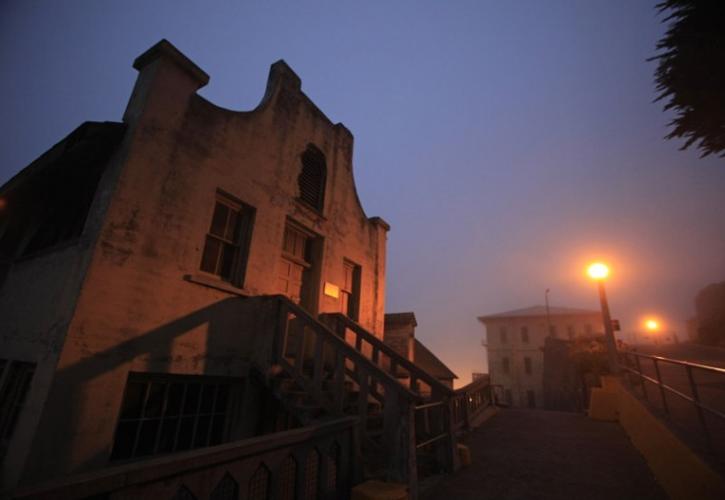The photograph is a rectangular image taken outdoors during the early evening hours, capturing a cityscape at dusk. Dominated by a muted color palette of blues, yellows, whites, blacks, and tans, the scene features two primary buildings of old, primitive architecture.

On the left side of the image stands an old stone building with a weathered façade, featuring two simple windows and a wooden door on the ground floor, and another window above the door. Leading up to the wooden door are a set of stairs with railings on both sides. Just beneath this building, a narrow walkway begins, featuring similar stone stairs and railings.

This walkway extends towards the bottom middle of the image, climbing slightly to connect with another, more distant three-story building positioned towards the right middle of the frame. This latter building, constructed of cement or plaster, appears deserted and has a metal plaque on its entrance door. A gate blocks entry to the stairway leading up to this building.

In front of this house, two streetlights mounted on metal posts illuminate the scene with a distinctive bright orange glow, contrasting against the deepening blue sky of dusk. The top right corner of the image hints at a small part of a tree, suggesting urban vegetation. The entire setting feels reminiscent of a non-US city, marked by unique architectural details and a quaint, almost historical ambiance.